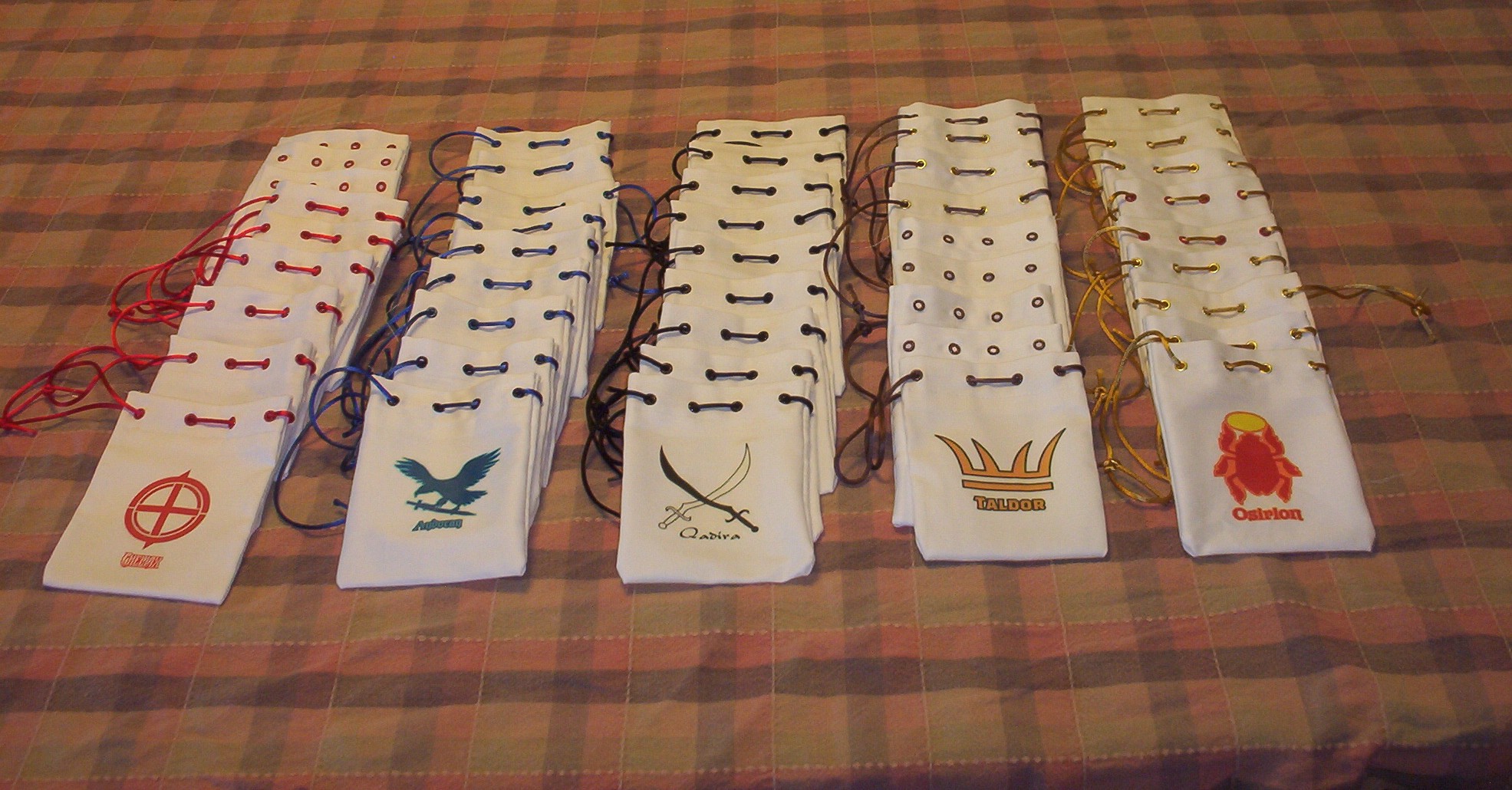The image depicts a collection of white drawstring bags arranged vertically in five columns on a brown plaid cloth with intricate designs in various shades of brown, dark green, and light brown. Each column features bags of a single design and color scheme. Starting from the left, the first column of bags has a red circle with a cross in the center, accompanied by illegible red writing and red drawstrings; the top three bags have red holes instead of laces. The second column showcases a blue silhouette of a crow holding a knife with blue writing underneath and blue drawstrings. The middle column displays two crossed swords, one black and one white, with the word "QADIRA" in black text beneath and black drawstrings. The fourth column features a gold crown with the word "TALDOR" in yellow text below and brown drawstrings. The rightmost column shows a red scarab with the text "OSIRION" below and gold drawstrings. The entire arrangement sits atop the themed cloth, providing a visually coherent yet detailed presentation.